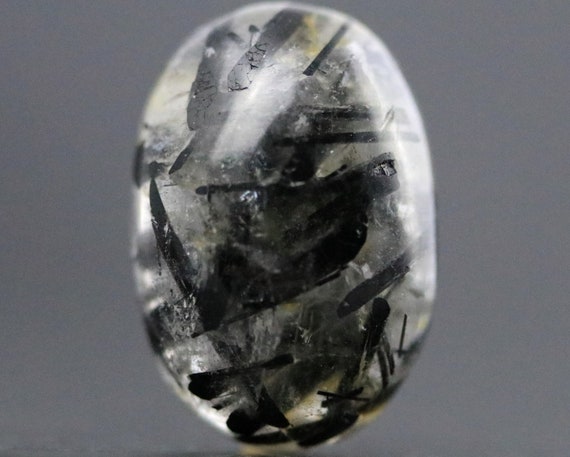This is an up-close view of an egg-shaped crystal, reminiscent of a Fabergé egg, featuring a polished, translucent surface. The background is a flat charcoal gray, providing a striking contrast. Inside the crystal, dark black lines, resembling brush strokes or ink streaks, criss-cross at sharp angles with varying thicknesses and directions. Some areas include yellow spots amidst the black streaks. The light source, coming from the top right of the photo, reflects off the glossy surface and also penetrates the translucent material, illuminating the black lines from within. Toward the bottom, the black embellishments—resembling carbon or graphite—are more concentrated and appear to touch the interior surface of the egg. At the top, some parts of the black lines show signs of wear, suggesting possible chipping or cracking in the paint or the crystal itself. The overall effect is a dynamic and intricate interplay of light and dark within the three-dimensional, egg-shaped structure.